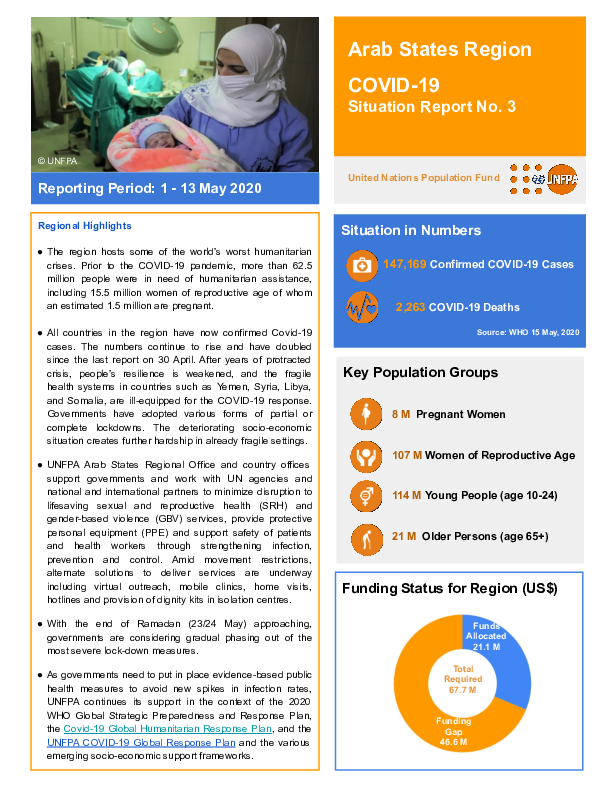This infographic on a white background with black text provides a detailed overview of the COVID-19 situation in the Arab States Region. The design is twice as tall as it is wide, featuring colored elements in blue and light yellowish-orange.

At the top left, a photograph shows a person in surgical scrubs and a white face covering holding a newborn swaddled in a pink and white blanket. Behind them, other medical professionals in blue surgical scrubs are gathered around an operating table, indicating a hospital or operating room environment.

The main text beneath the photograph reads "Reporting Period: 1-13 May 2020." Below this, a boxed-in bulleted list of regional highlights is outlined in orange, providing key updates and information.

On the right side of the infographic, an orange box at the top reads "Arab States Region COVID-19 Situation Report No. 3." This is followed by sections including a blue box with "Situation in Numbers," a gray box titled "Key Population Groups," and a white box detailing the "Funding Status for the Region in U.S. Dollars." The funding status section also includes a pie chart with yellow and blue segments, visually representing the funding distribution.

The infographic combines visual data representations and textual information to provide a comprehensive overview of the COVID-19 situation in the specified region during the reporting period.